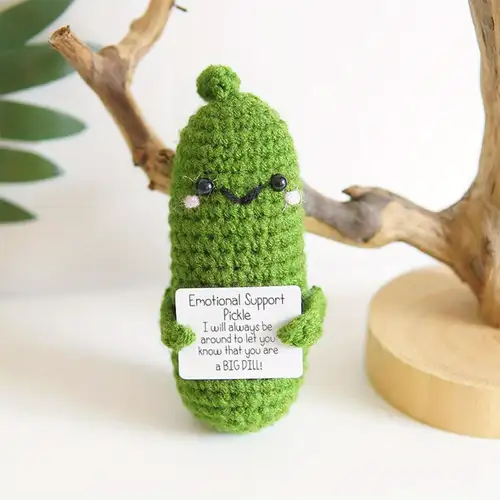In the center of the image, there is a knitted toy shaped like a pickle, featuring small black eyes, a yarn smile, and two white dots on its cheeks. The green pickle has tiny arms holding a white sign that reads: "Emotional Support Pickle. I will always be around to let you know that you are a Big Dill." The text "Big Dill" is emphasized with capital letters. The pickle is positioned on a wooden platform against a white wall backdrop. To the right, there is a jagged branch extending into the scene, while to the left, green leaves from a plant are visible. The overall setting conveys a cozy, supportive atmosphere with the whimsical stuffed toy as the focal point.